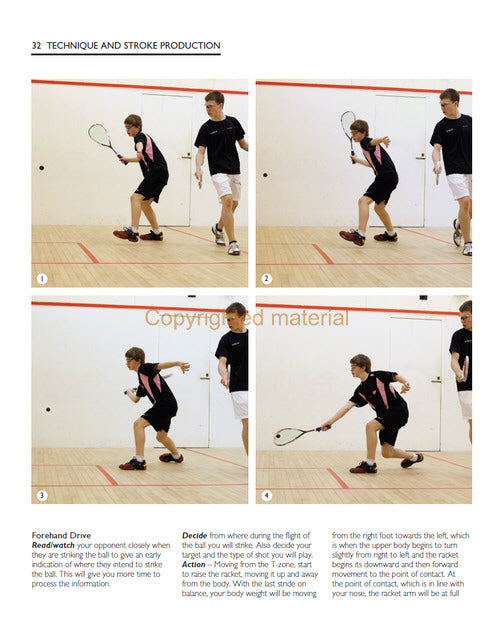This appears to be a textbook page on how to play pickleball, specifically focusing on technique and stroke production as indicated by the heading "32 Technique and Stroke Production" at the top. The page features four sequential photos showcasing two teenage white males practicing a forehand drive. The boy in the black shirt and black shorts is shown in various stages of executing a swing with his racket, targeting a ball that progressively approaches him in each image. Meanwhile, another boy wearing a black shirt and white shorts stands nearby, possibly acting as an opponent or partner.

The instructional text beneath the photos emphasizes the key steps for a proper forehand drive. It advises the reader to closely observe the opponent’s movements to predict where the opponent will strike the ball, allowing more time to plan their own shot. It then outlines the action steps: starting with positioning in the T-zone, raising the racket up and away from the body, transferring body weight from the right foot to the left, and rotating the upper body from right to left as the racket descends and moves forward to hit the ball at the point of contact, which should align with the nose. The racket arm should be fully extended at this point. The page also includes a note indicating that the content is copyrighted material.

Overall, the visual and textual information provides comprehensive instructions on the forehand drive, illustrating the detailed steps involved in executing this technique properly.